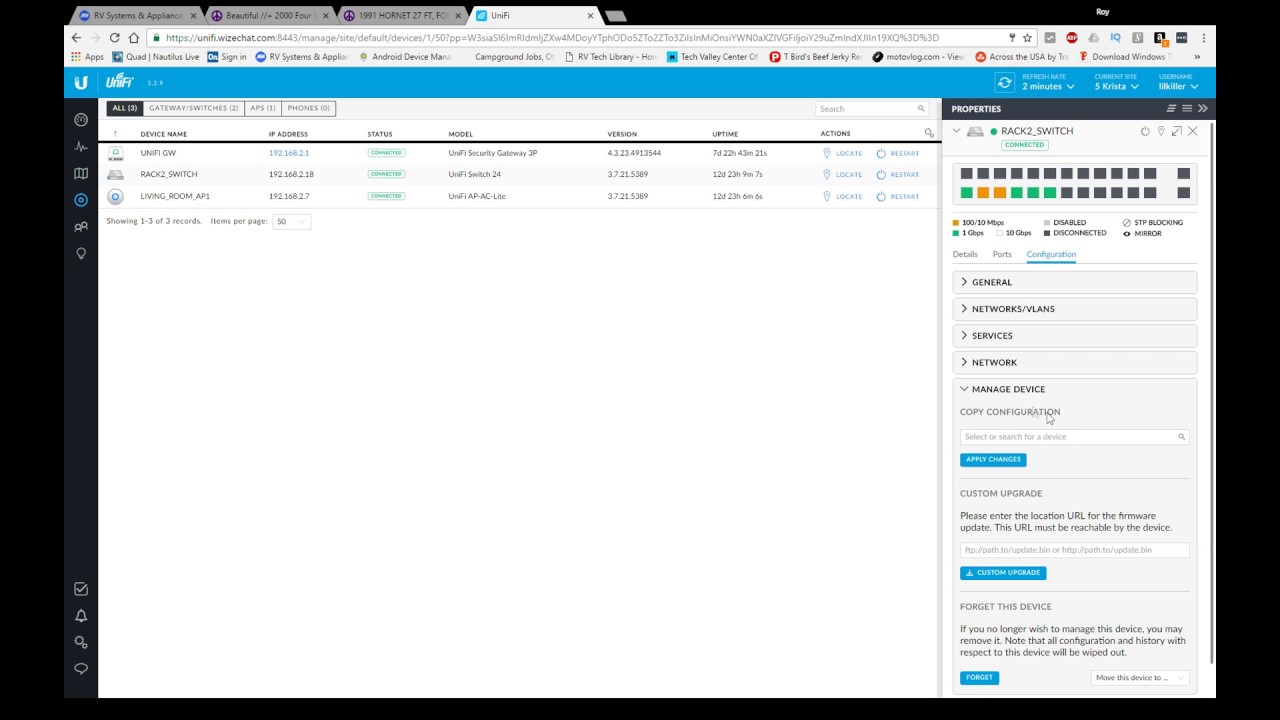This screenshot captures the dashboard of a platform named "Unify," which appears to manage and control various smart devices. The interface, accessible via a URL beginning with unify.wisechat.com, prominently features a layout reminiscent of a file storage system. However, a closer examination reveals its function as a device management hub.

In the main section of the dashboard, three devices are listed: Unify GW, Rack2Switch, and Living Room AP1. Each device entry includes detailed information such as their respective IP addresses, current connection statuses (all marked as connected), device models, software versions, and uptimes, indicating how long each has been operational. Users have control options at their disposal for each device, including locating and restarting them.

Currently, the device labeled "Rack2Switch" is selected, as evidenced by a property panel displayed on the right-hand side of the interface. This panel provides in-depth properties specific to the Rack2Switch device, offering further insights and management capabilities.

In the upper left corner of the dashboard, the Unify logo and name are clearly visible, emphasizing the brand of the platform. Despite the text being somewhat difficult to read, zooming in allows for a better view of these elements. This structured and detailed layout underscores the platform's utility in overseeing a network of interconnected devices efficiently.